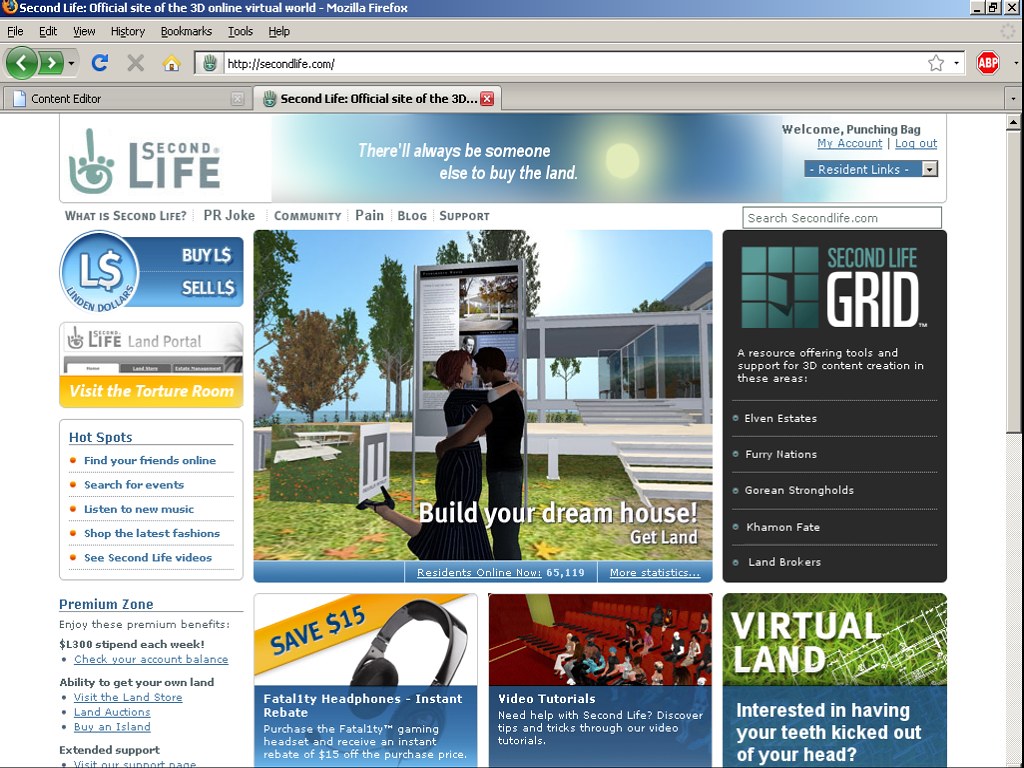This is a detailed screenshot of a web page displayed in a Mozilla Firefox browser. At the top, the Firefox logo is on the left side of a blue gradient bar that transitions from dark to light blue, alongside the title "Second Life, official site of the 3D Online Virtual World - Mozilla Firefox." The window control buttons for minimize, maximize, and close are on the upper right corner. Below this, the traditional menu bar includes options like File, Edit, View, History, Bookmarks, Tools, and Help. The navigation toolbar features green back and forward buttons, a blue reload button, a gray (disabled) stop button, and a home button depicting a house with a yellow roof. The address bar shows "http://secondlife.com," and two tabs are open: one labeled "Content Editor" and the other active tab titled "Second Life, official site of the 3D Online Virtual World."

The webpage content has a large banner displaying "Second Life," with a sun icon emitting yellow rays on the upper right. Text next to it reads, "There will always be someone else to buy the land.” The page greets the user as "Welcome PunchingBag" and provides links for "My Account" and "Logout," followed by a drop-down menu for resident links. Additional navigation tabs include "What is Second Life," "PR Joke," "Community," "Pain Blog," and "Support."

A prominent image at the center of the page shows two computer-generated characters embracing in front of a futuristic house, accompanied by the text "Build your dream house, get land." Below the image, a section indicates "Residents online now: 65/119," with more detailed statistics available.

The left side of the page showcases various sections and ads, including "Buy L$", "Sell L$", "Land Portal," "Hotspots," "Find your friends online," and "Search for events." Ads for products and services, such as "Fatality Headphones," "Instant Rebate," video tutorials, and advertisements for virtual land opportunities, are also prominent. The right-hand side includes another detailed navigation section under "Second Life Grid," highlighting resources and support for 3D content creation, with links to "Elvin Estates," "Furry Nations," "Gorean Strongholds," and more. The page also features standard vertical scroll bars for navigation.